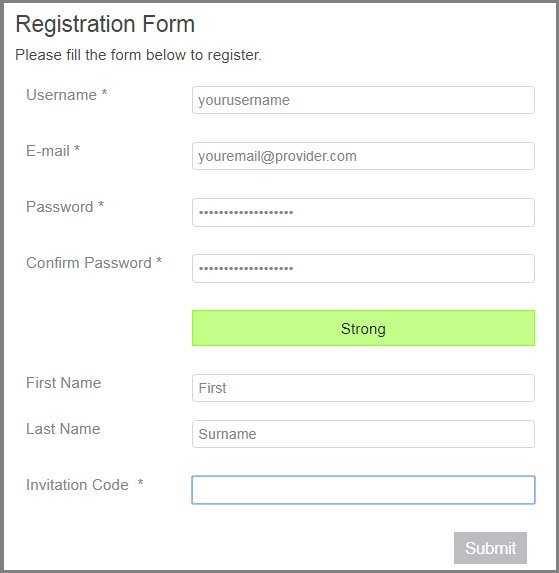The image depicts a registration form, intended for online use, featuring a clean and straightforward design. The form heading reads "Registration Form" in dark, bold text, instructing users to "Please fill in the form below to register." The background is predominantly white, with subtle gray boxes indicating the fields to be filled.

Starting from the top, the form requests a "Username," with a note to the right clarifying, "Your Username," specifying what the user should input. The next line is for the "Email," accompanied by a placeholder example, "your email at provider.com," to guide users on the format required.

Following the email section, there are fields for "Password" and "Confirm Password." An indicator appears to assess the password strength as "Strong," providing feedback on the password's adequacy.

The form continues with fields for "First Name" (noted as "First" after the field) and "Last Name" (noted as "Surname"). There is also an "Invitation Code" field, which remains blank, suggesting it is optional or to be filled if the user has a specific code.

All instructional and field-label texts are in a dark color to ensure readability against the white background. As the form visually guides the user through the registration process, it emphasizes the importance of a strong password and provides clear input examples, enhancing user experience and minimizing input errors.